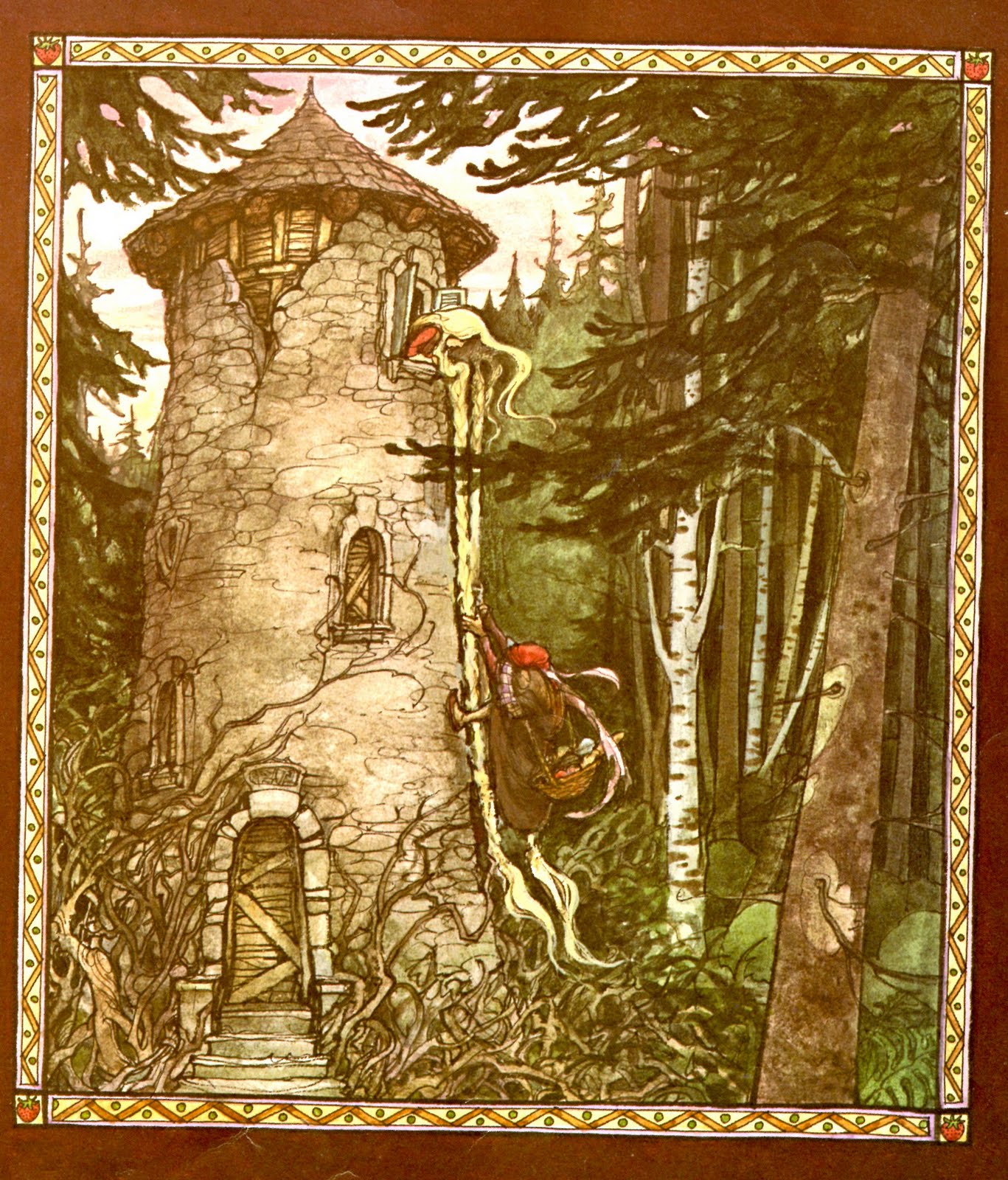The illustration, a book plate from the fairy tale Rapunzel, depicts an elaborate, cartoonish scene set in a heavily wooded forest. The focal point of the image is a tall, decaying stone tower with a distinctive mushroom-shaped roof. The tower is adorned with cracked stones, dead vines, and some exposed foundation, lending it an aged and weathered appearance. On the right-hand side near the top, a set of window shutters is open, and Rapunzel, a woman with long, blonde hair braided into two separate strands, leans out of the upper window. Her red dress stands out vividly against the somber tones of the building. Her hair streams down the entire height of the tower, almost touching the ground.

Climbing up Rapunzel's hair is the prince, characterized by his rather obese figure, brown cape, and a distinctive red cap. He has a rope slung over his shoulder and carries a basket on his back, filled with indistinguishable items. The prince is using both his hands and feet to grip the braided hair as he ascends, approximately halfway up the tower. Surrounding the base of the tower are dense brambles, roots, and vines, contributing to the forest's overgrown and untamed feel. The scene is framed by tall trees, some white and some brown, consistent with a mix of pine and other species. The entire illustration is encompassed by a decorative gold frame, enhancing its fairy tale charm and setting a magical tone for this classic story retelling.